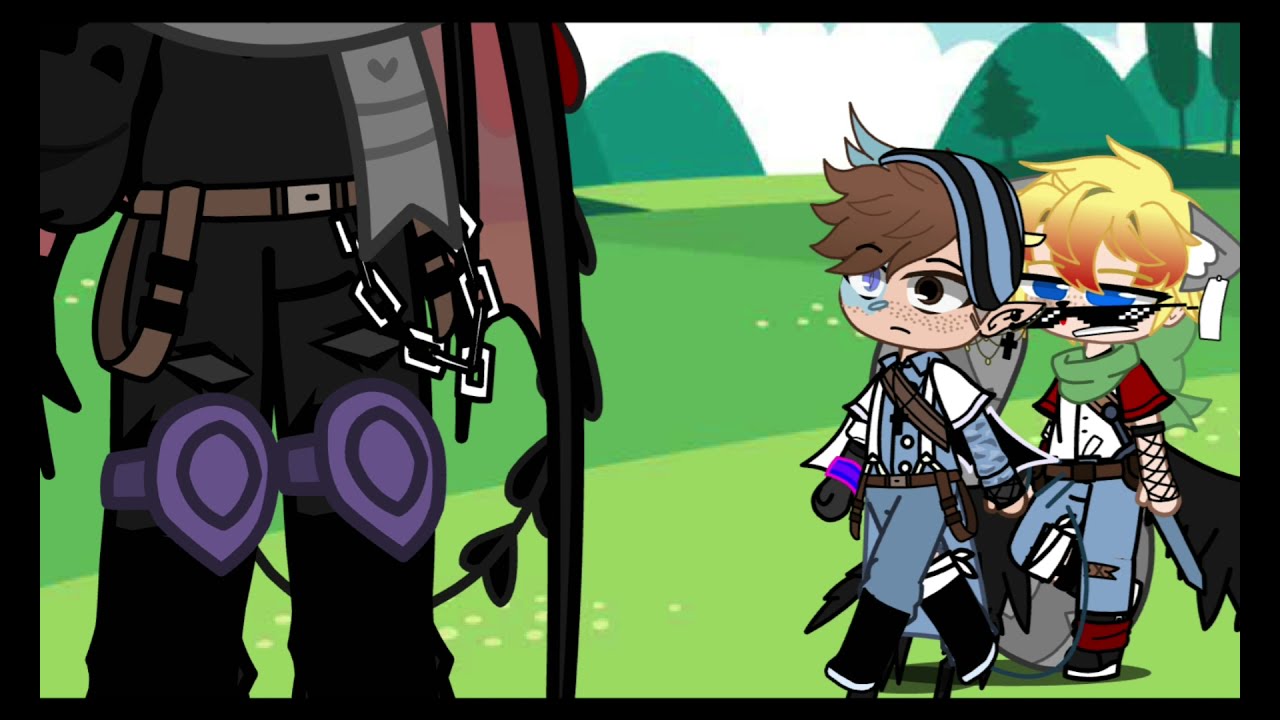In this cartoon animation set in a landscape layout, there are three distinct characters. On the right side, there are two young people walking together. The person in front has brown hair with a light blue and black striped fabric on top, possibly a beanie. They have one purple eye, one black eye, and light peach skin with freckles. They are dressed in a light blue suit with black shoes, and a backpack. Just behind them is a second person with yellow and orange hair, wearing sunglasses with black frames, a white shirt, blue pants, a green scarf, and a black cape. They also have red accents on their shoulders and around one ankle. On the left side of the image, the legs and lower torso of a figure dressed in black with purple knee pads are visible. This figure has a brown belt with a lighter brown central section and a chain hanging from it. The background features a green field with varying shades of green, rolling hills, and white clouds with ripples. Two trees are visible in the upper right corner, and there's a reflection of a pine tree on one of the hills. The entire scene is bordered in black, enhancing the cartoonish, fantasy adventure vibe of the image.